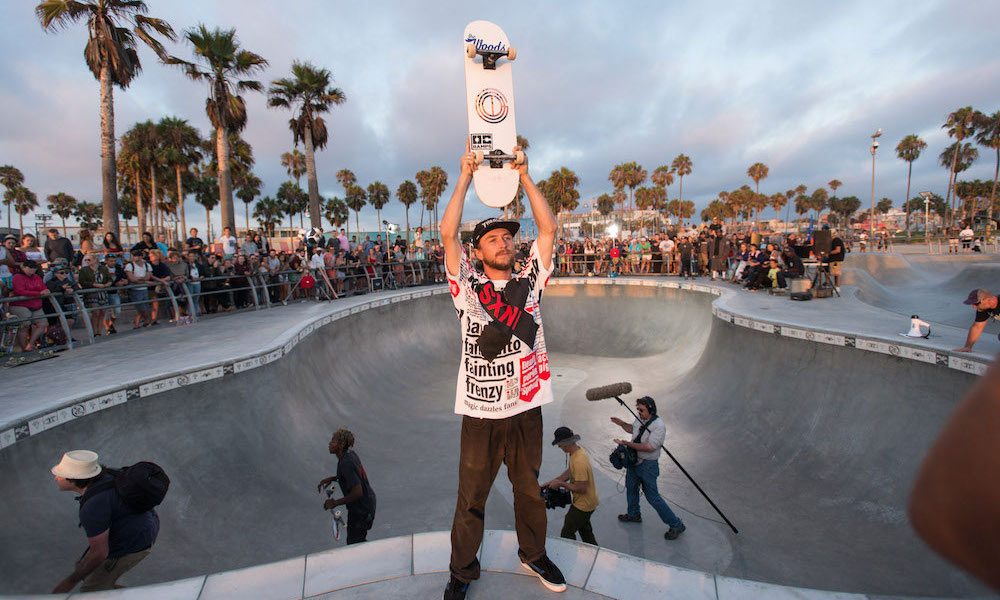The image captures a vibrant skateboarding event, set in an empty swimming pool repurposed as a skate bowl with gray concrete forming a unique triangular shape with three semicircular areas. In the foreground stands a young man, likely in his 20s, wearing a black baseball cap, a white shirt adorned with black and red designs resembling a tabloid print, brown pants, and black and white sneakers. He's hoisting a white skateboard vertically above his head in a celebratory pose, both arms extended. Around his neck is a black scarf emblazoned with the letters "SXN."

Within the skate bowl, there are a few skateboarders and a film crew comprising three white men and an African-American youth. The African-American skater sports a black shirt and pants, while another skateboarder wears a blue shirt, white hat, and brown pants. The film crew is equipped with a boom mic and a camera, indicating they are capturing footage of the event.

Encircling the skate bowl is a low, metal guardrail behind which hundreds of spectators have gathered to watch the action. The backdrop features rows of tall palm trees, suggesting the location is likely in California or Florida. The sky above is a light gray with hints of pinkish-gray clouds, adding an atmospheric touch to this lively scene.